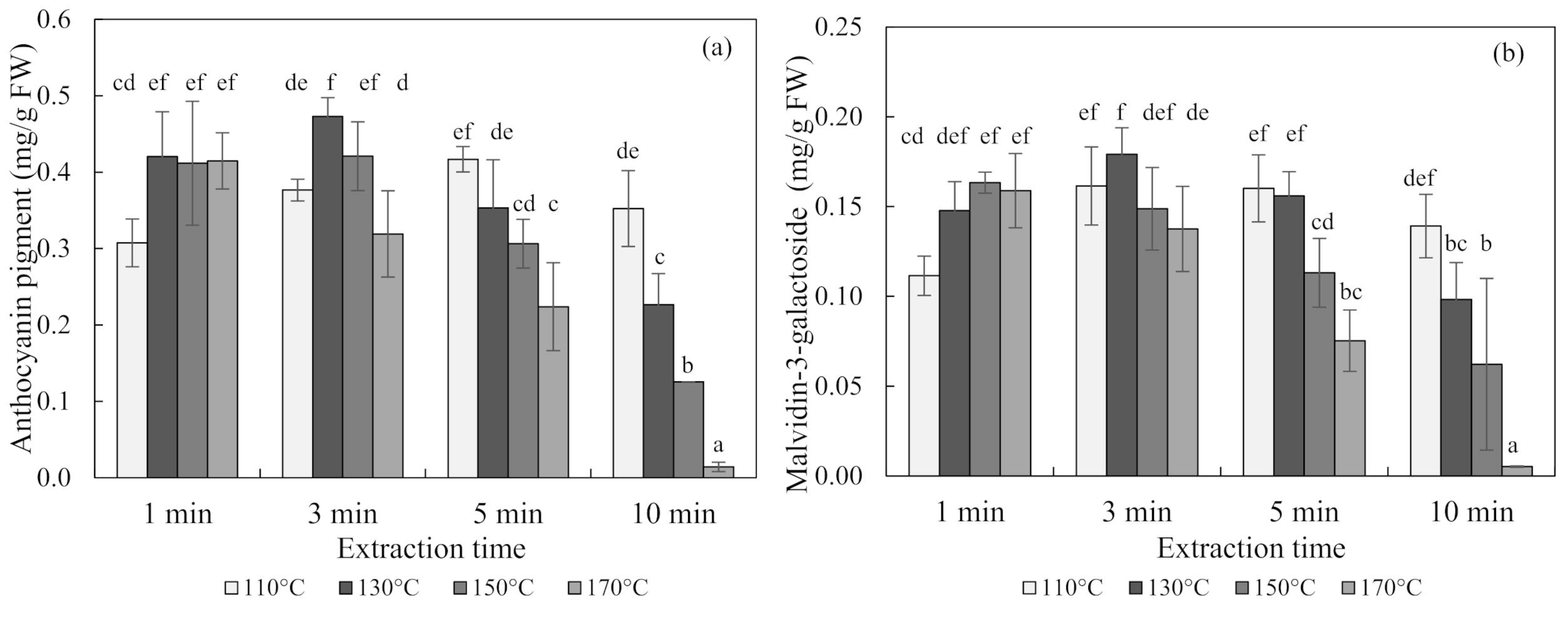The image consists of two black-and-white bar charts arranged side by side, each displaying data over identical time intervals and temperature conditions. The left chart illustrates the "Anthocyanin Pigment" concentration in milligrams per gram of fresh weight (mg/g FW) and is labeled from 0.0 to 0.6 on the vertical axis. The right chart shows the concentration of "Malvidin-3-Galactoside" in mg/g FW, scaled from 0.0 to 0.25. Both charts have the horizontal axis divided into 1-minute, 3-minute, 5-minute, and 10-minute intervals and feature bars representing temperatures of 110°C, 130°C, 150°C, and 170°C in varying shades of gray—light gray for 110°C, medium gray for 130°C, darker gray for 150°C, and the lightest gray for 170°C. Each time interval features four bars corresponding to these temperatures. Above the bars, letters indicate specific statistical groupings such as CD, EF, EF, EF on the left chart, and DECBA, and others on the right chart.